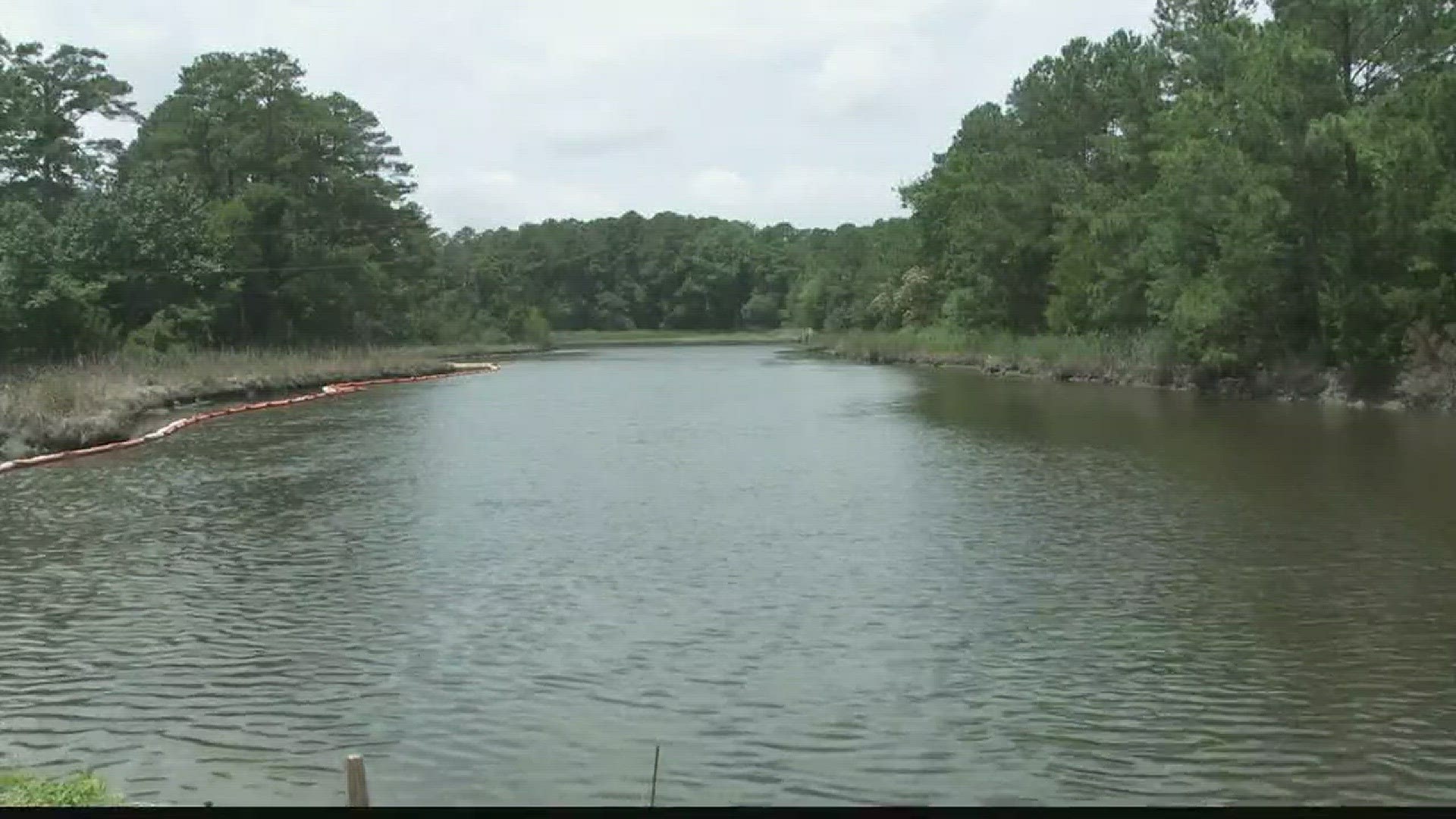The image depicts a serene, greenish lake surrounded by a dense forest. The water, tinged with green from possible algae or murkiness, extends across the lower third of the image, creating subtle ripples. The shoreline is lined with lush grasses and weeds, with no sandy beaches in sight. To the left and right, as well as in the distance, tall green trees densely populate the area, contributing to the image's secluded and tranquil atmosphere. The sky above is cloudy and overcast, adding a moody ambiance but with no signs of rain. The image includes some indistinct lighter colored strip on the left shoreline and some rocks on the right, but no human presence is noted. The scene captures a peaceful, natural environment with a harmonious blend of water and forest.